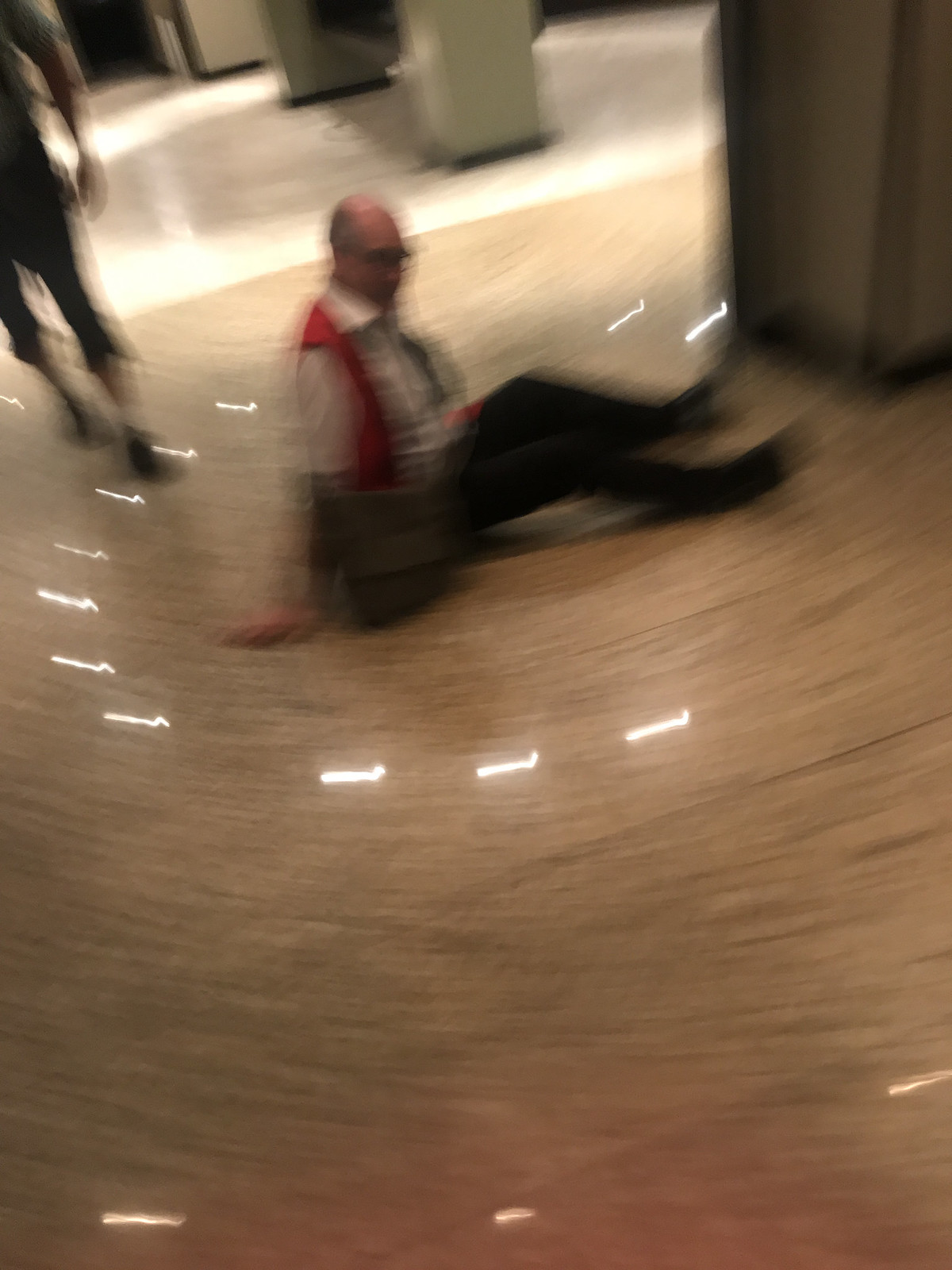A man is sitting on a glossy granite floor with his knees up, wearing dark pants, a short-sleeved white collared shirt, a red vest, and glasses. His hands are resting on the floor, suggesting he might be about to stand up. Reflections of overhead lights shimmering on the floor add a slight blur to the scene. In the background, a partially visible person is walking away, with only their legs discernible. Pillars elegantly stand in the distance, completing the composition.